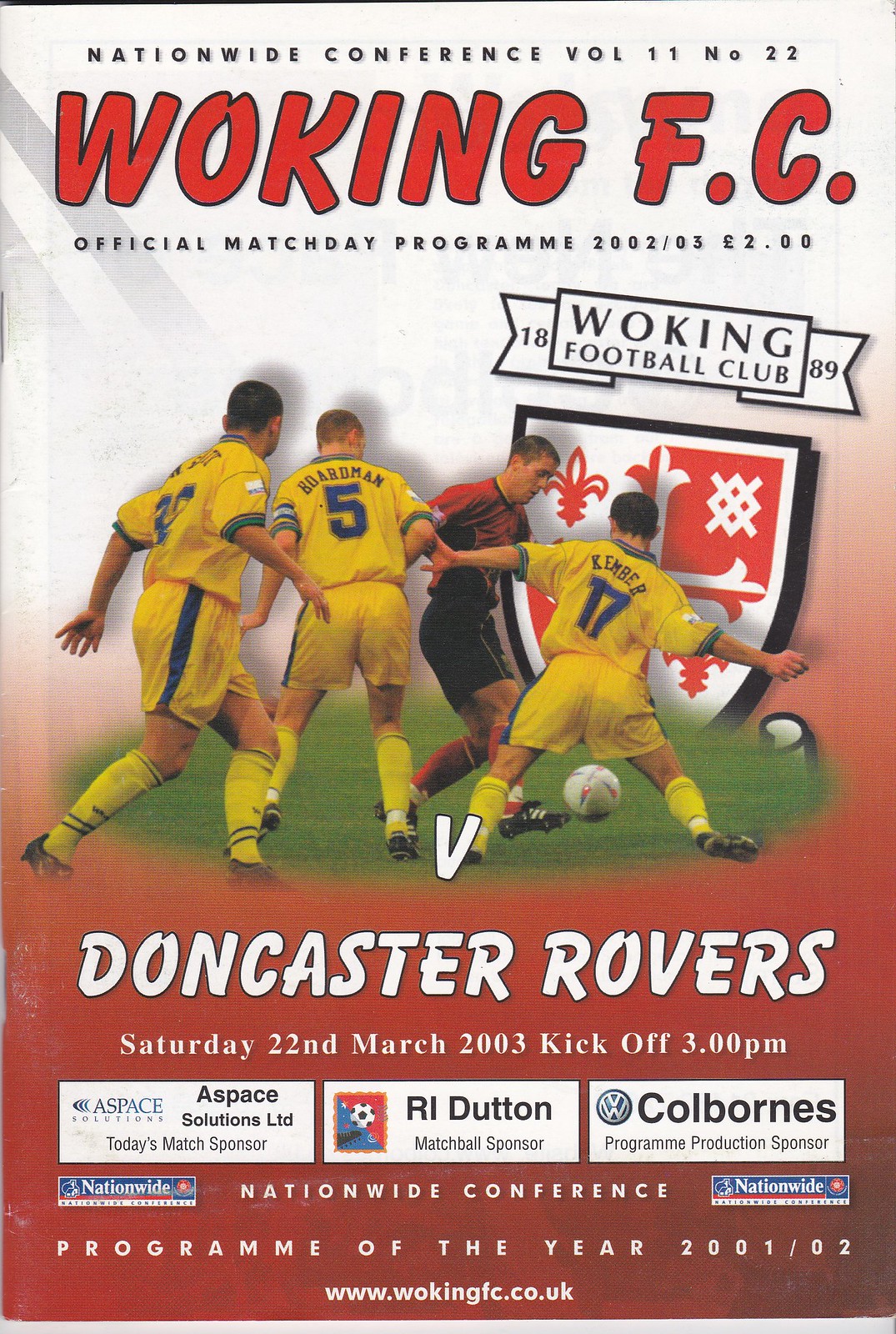This detailed description pertains to an official match day program for Woking FC versus Doncaster Rovers held on Saturday, March 22, 2003, with a kickoff at 3 p.m., part of the Nationwide Conference. The top portion of the program, predominantly white with black text, reads "Nationwide Conference, Volume 11, Number 22." Below, in red, it states "Woking FC Official Match Day Program 2002-03," priced at two pounds. Just beneath this, a white banner in black text heralds "Woking Football Club, 1889." Central to the design is a graphic image featuring football players: two in yellow jerseys with blue numbers, yellow socks, and black shoes, numbered 5 and 17, and one opponent in a red jersey and black shorts with red socks. Positioned along the bottom, a red strip highlights various advertisements including sponsors like Aspace, RI Dutton, and Colborne's Volkswagen. Additionally, the program proudly announces its accolade as the "Nationwide Conference Program of the Year 2001-02," with the club's website: www.wokingfc.co.uk.